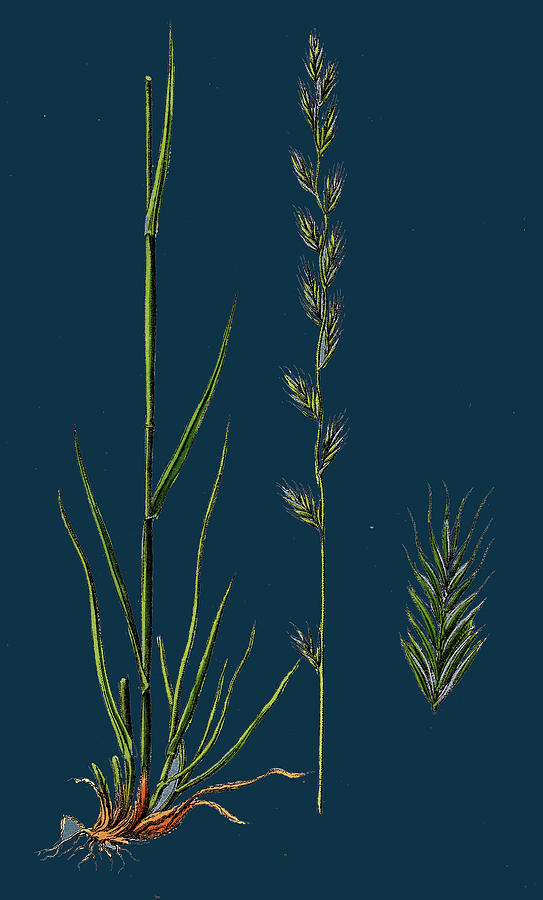A detailed painting features a botanical scene set against a dark blue, night sky-like background with subtle hints of green. The central composition highlights three distinct plant elements. On the left, there is a tall, bamboo-like stem showing vibrant orange roots at the base and twisting, slender green leaves climbing upwards. In the middle, a stalk reminiscent of wheat displays fluffy leaves and spiky projections, giving the appearance of a slender, elongated flower with tiny feathery blossoms adorning its length. On the right, a magnified view of one of these feathery blossoms showcases intricate details of its structure, emphasizing its delicate, wispy projections. This intricate arrangement, without any textual context, offers a vivid portrayal of different botanical forms and their unique textures.